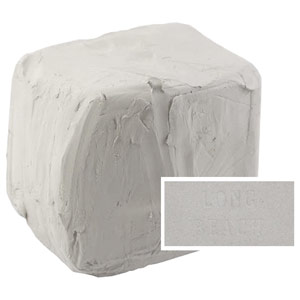The image depicts a white or pale grayish block of clay, irregularly shaped, not a perfect cube but more of a rough, squarish form with some sides appearing smoother than others. Visible cut or chipped areas suggest pieces have been removed. The clay block is placed against a white background that accentuates its color, or rather its lack of vibrant color. A small square inset, which looks like a zoomed-in section of the block, features a white border and the text "Long Beach," although the significance is unclear. The inset suggests a focus on this textual detail within the larger context of the clay block.